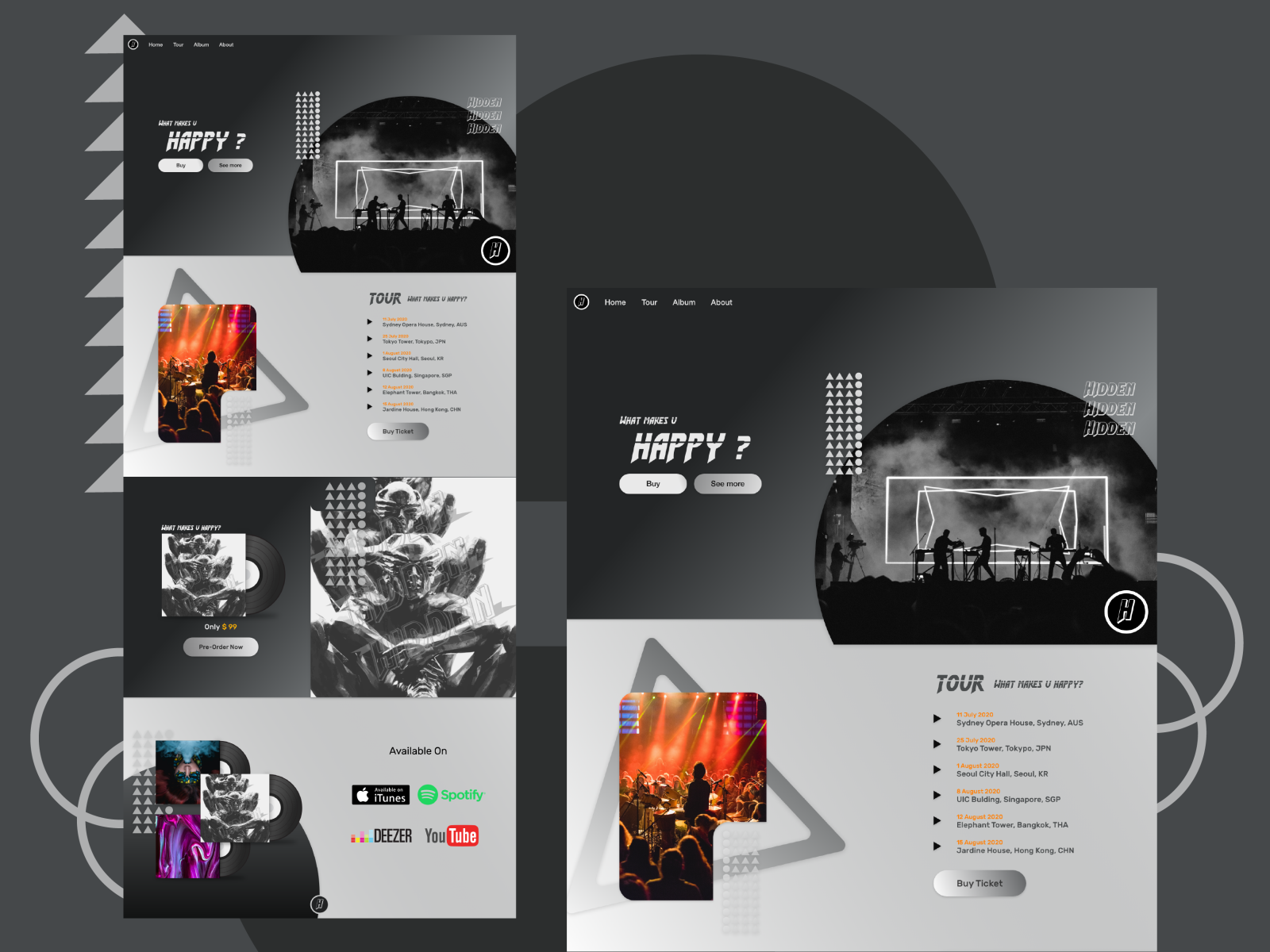A detailed screenshot depicts a promotional web page for a music band. The predominant background color is various shades of gray, with some sections featuring lighter gray triangular shapes and a darker gray circular element in the backdrop. The central portion of the image prominently displays a query: "What makes you happy?" followed by interactive options to "buy" or "see more."

Midway through the screen, an image of the band performing on stage is visible, overlaid with the repeated word "hidden." Below this, the webpage announces the band's tour with the slogan "What makes you happy" followed by an abbreviation "4 U."

Further down, the page provides details about ticket purchases and features a section hinting at the band members' identities. The record is available for pre-order at the price of $99, as indicated by the text "Pre-order now." Additionally, the availability of the album on various streaming platforms is noted, including Apple iTunes, Spotify, Deezer, and YouTube. Surrounding these details are various images of the band performing live on stage, contained within gray boxes.